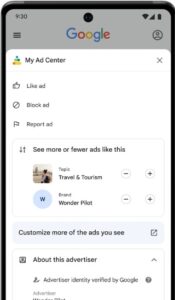The image depicts a smartphone displaying a screen from Google's interface. The phone has a black outline and a gray area at the top where the time is shown as 9:30 on the upper left corner. On the upper right corner, icons for Wi-Fi signal strength and battery status are visible. 

At the center of the screen, the word "Google" is prominently displayed. Below that, a pop-up window titled "My Ad Center" appears in the upper left corner with an "X" on the upper right corner to close it.

The pop-up features three interactive options presented vertically:
1. A thumbs-up icon labeled "Like Ad."
2. A circle with a line through it labeled "Block Ad."
3. A flag icon labeled "Report Ad."

Further down, there is a box with an up and down arrow on the left labeled "See More or Fewer Ads like this." 

Below this section, two specific ad categories are shown:
1. "Travel and Tourism" accompanied by an image of a person outdoors.
2. "Wonder Pilot," represented by a blue circle with a "W" inside it.

At the bottom, a light blue button prompts users to "Customize More of the ads you see."

Finally, a white box at the very bottom of the screen contains the title "About This Advertiser," with a note that states, "Advertiser Identity Verified by Google."